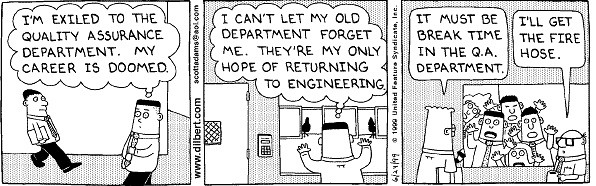This is a black and white, three-panel comic strip from Dilbert.com dated 06-24-1999. Each panel, equal in size, humorously depicts an office setting with characters in dress pants, ties, and shirts. In the first panel, two people walk around an office, with one saying, "I'm excited. I'm exiled to the quality assurance department. My career is doomed." The second panel shows a man peeking through windows at people sitting inside, stating, "I can't let my old department forget me. They're my only hope of returning to engineering." The final panel features a crowd of people staring through a window at the engineering department, with one insider remarking, "It must be break time in the QA department. I'll get the fire hose."